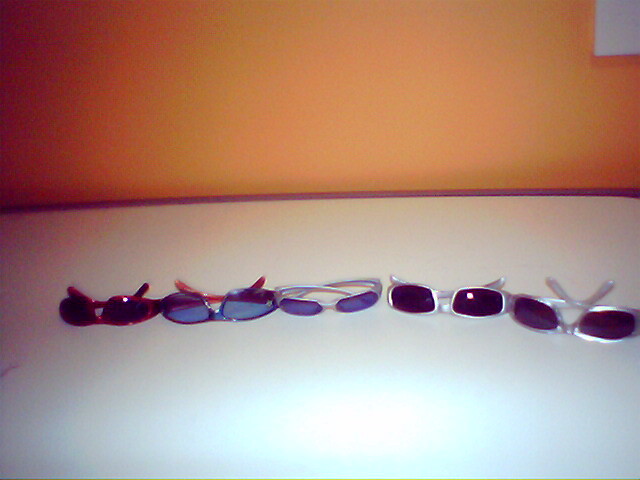This indoor color photograph captures a close-up of five pairs of sunglasses arranged in a row on a white surface, possibly a seat or counter. The background features an orange wall, adding a warm hue to the scene. The sunglasses are displayed upside down on the tops of their frames, with the earpieces sticking up and occasionally crossed behind. Each pair showcases a variety of frame colors and lens types: red frames with black lenses, black frames with grayish lenses and red inner arms, two silver frames with purple lenses, and a clear frame with dark lenses. The arrangement is meticulous, displaying different shades and styles, including wraparound and rectangular shapes. Despite some glare from the flash, the details of the crossed arms and the diverse colors and designs of the sunglasses are clearly visible.